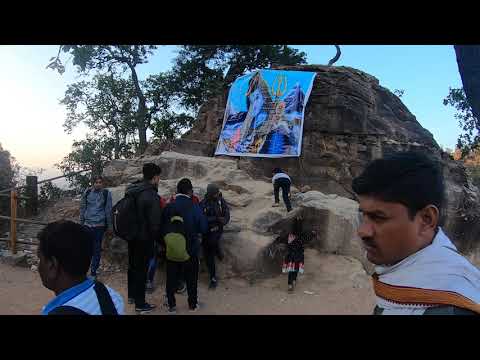This detailed photograph captures a diverse group of people gathered around an imposing rock formation set in a sandy landscape. The rock formation has a dome-like shape with a lighter beige lower section transitioning to a darker brownish-gray top. Draped from the top of the rock, a large, colorful poster, reminiscent of a blanket, hangs prominently. The poster is vibrantly colored with hues of blue, gold, gray, brown, and pink, depicting a scene that the observers seem to be studying closely. 

In the foreground, a boy is seen climbing the beige section of the rock, his small figure contrasted against the imposing formation. Surrounding the rock, several individuals dressed in warm clothing—sweatshirts and long pants—are clustered. One man, with dark hair, mustache, and dark skin, dressed in a white and gold garment, stands prominently to the right, his profile visible. Another man, nearby, with even darker skin and wearing a blue-collared white shirt, appears to be walking by. In the background, trees dot the landscape, adding a natural frame to the scene.

The image, bound by thin black bars at the top and bottom, appears to be a still taken from a video, adding a cinematic quality to the moment captured. The overall scene is set against a backdrop of white and blue skies, creating a striking contrast between the natural elements and human activity.